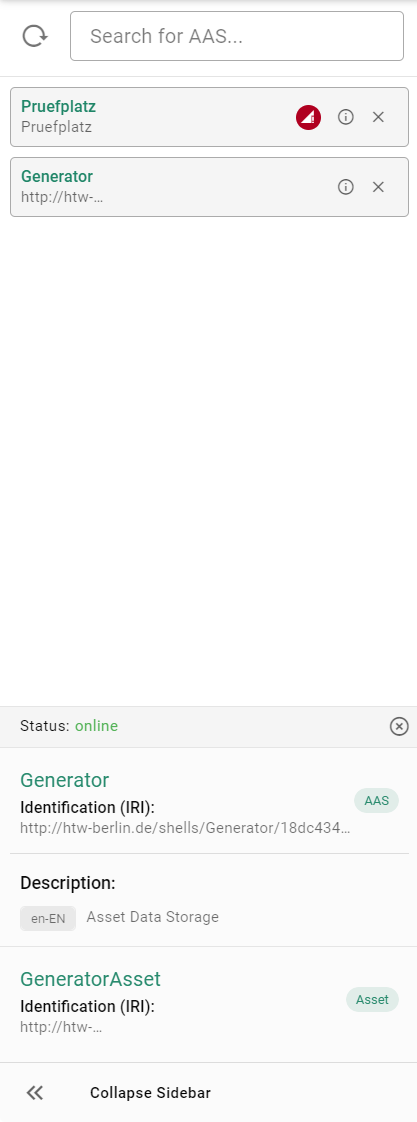A screenshot of a website displayed on a phone with various technical terminologies and icons.

At the top of the screenshot, there is a search bar that prompts users to "search for AAS..." Below the search bar, there is a word that appears to be in German: "Prüfplatz." This word is displayed prominently in green text. Adjacent to it, the same word appears in standard black text. Next to the black text are three icons on a light grey background: a red circle containing a small white triangle pointing upwards, a white circle with an 'i' inside, and a red circle with a white cross.

Further down, the word "generator" is again displayed in green text followed by a fragment of a web address starting with "http://htw..." but it is incomplete. No red circle is present here, only an icon similar to the 'i' in a circle with a cross.

A large blank space appears underneath these details, followed by additional messages. The word "status" is shown in regular text with "online" next to it, indicating a successfully running status. The next segment mentions "generator identification (IRI)" and lists a more complete URL: "http://htw-berlin.de/shells/generator." 

A green button labeled "AAS" is shown below this, alongside the word "description," and an option marked with "ENEN" which likely refers to selecting the English language. Lastly, several terms related to assets are mentioned, such as "asset data storage," and "generator asset identification."

Overall, while specific meanings and functionalities are unclear, the screenshot appears to belong to a technical or engineering-oriented webpage, possibly detailing information about specific assets or generators, complete with interactive buttons and multilingual options.